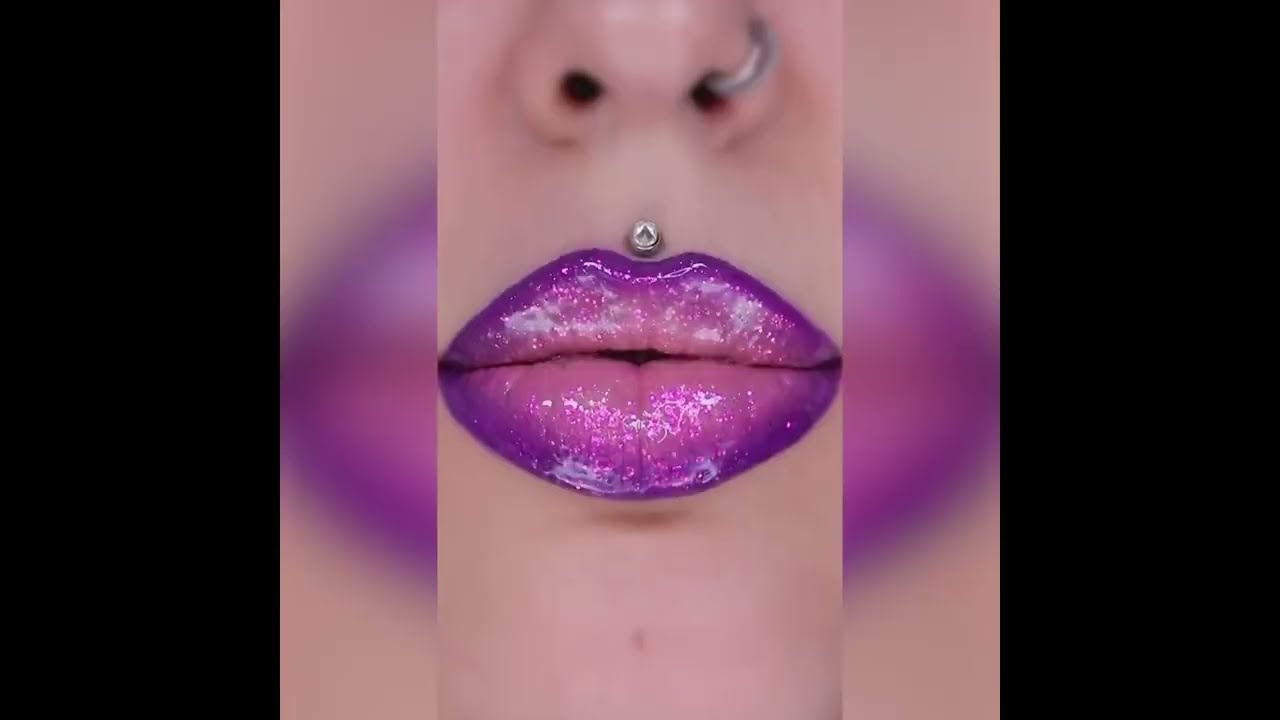The image is a three-sectioned photograph framed by thick black borders on the left and right sides. The central section features a close-up of a woman's lips adorned with purple, sparkly lip gloss that has a pinkish hue and a darker, lined outline. Her lips are closed, and just above her upper lip, there is a small circular metal stud piercing. The lower part of her nose is visible, featuring a silver ring in her left nostril. The top of her chin is also seen before the image cuts off. Flanking this central image are two blurry sections on the left and right, showing enlarged, out-of-focus portions of her mouth.